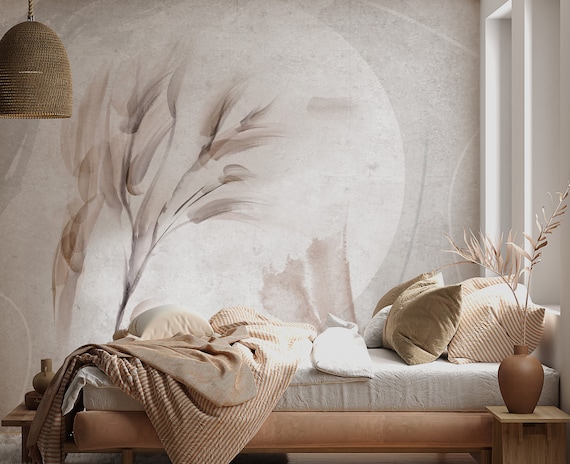The image showcases a serene, neutral-toned bedroom with a strong emphasis on beige and light grays. The bed, positioned with its headboard to the bottom right and footboard to the bottom left, features a white mattress topped with beige blankets and a mix of beige and white pillows. At the foot of the bed sits a beige bench, adding to the monochromatic theme. The walls are light gray, adorned with a large, decorative element that resembles a mural or wallpaper depicting beige leaves on branches. This natural motif is echoed by a wicker or straw-thatched hanging lamp suspended from the ceiling. A nightstand beside the bed holds a light brown vase with fronds or leaves, further amplifying the room's earthy and minimalist aesthetic. Additionally, a small wooden table with beige decorative objects is positioned near the headboard. The overall atmosphere is one of calm and simplicity, with well-coordinated natural elements and muted tones.